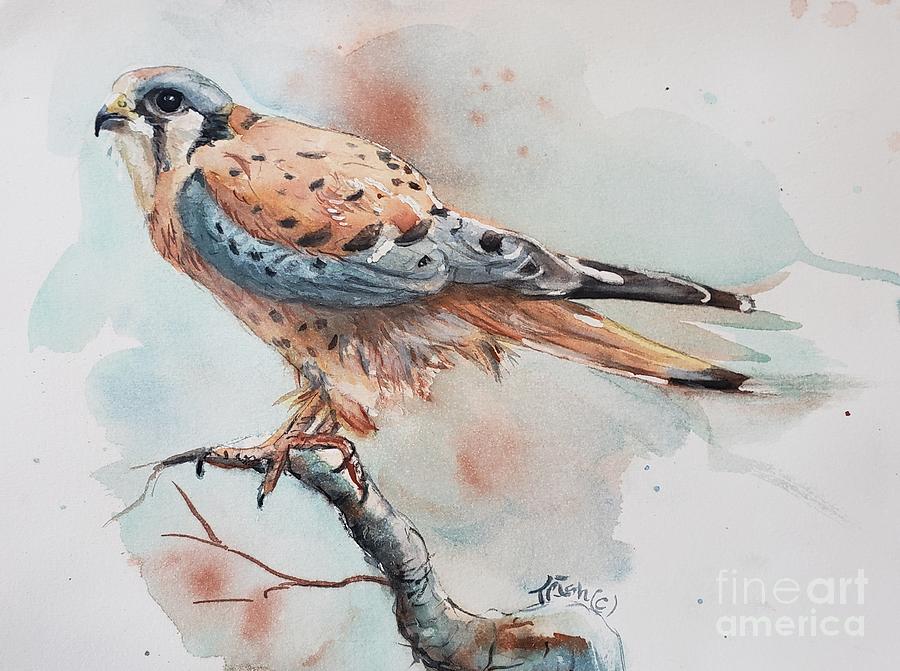This detailed watercolor illustration features a bird perched majestically on a single tree branch, which extends out of the frame. The bird, possibly a hawk or falcon, is depicted in side profile, looking to the left with one large, prominently grasping claw on the branch. Its feathers display a rich tapestry of colors, including browns, blues, blacks, light and dark oranges, grays, and speckles of black scattered throughout. The head is adorned with blue and brown hues, while its beak is short, stout, and tinged with yellow. The bird's piercing eye, rendered in inky black and the only one visible, adds to its keen expression. The loosely rendered yet detailed background employs a harmonious blend of blues, browns, reds, and purples, which combine to create an atmospheric setting for our feathered subject. In the bottom right corner, the words "Fine Art America" appear in white lowercase letters, and alongside this is a signature that reads "Trish" with a "C" in parentheses, completing this evocative illustration.